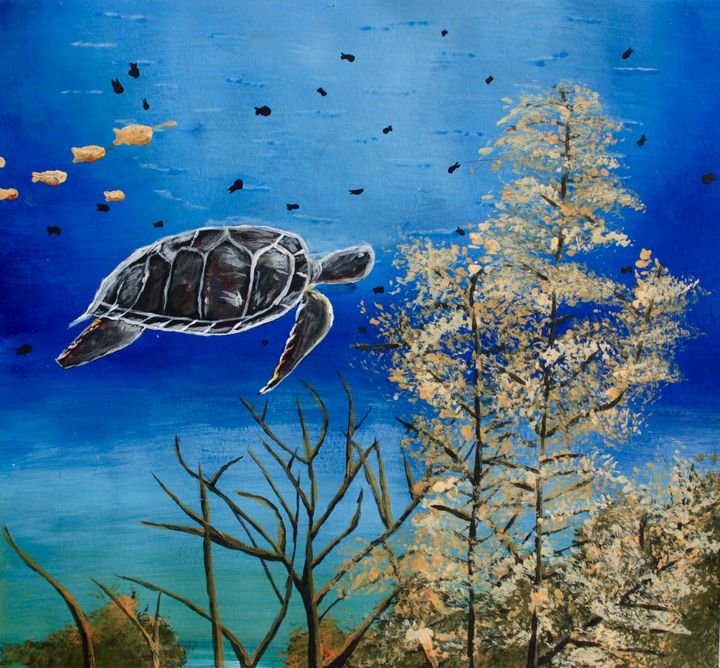This image appears to be an illustrated underwater scene reminiscent of a children's book. The painting is rich in aquatic details, featuring a serene, magical underwater world. At the center of the scene, a large sea turtle, dark green with a shell that almost appears greenish-black, swims gracefully to the right. His form is outlined in white, making him stand out against the varied hues of blue in the background. Surrounding the turtle, a small school of five orange fish also swim to the right, adding vibrant contrast to the scene. 

The ocean is illustrated with layers of blue, starting with a lighter blue near the surface that transitions into a darker blue as it goes deeper. Behind the turtle and the orange fish, a multitude of small, shadowy black fish can be seen, adding depth and a sense of bustling underwater life. Scattered across the sea floor are various types of marine plants; long, spiny plants with orangish-yellow leaves grow amidst a mix of seaweed and algae. These underwater plants, some just bare sticks and others full of life, add to the rich texture and detail of the painting, making it a vivid portrayal of the ocean's natural beauty.